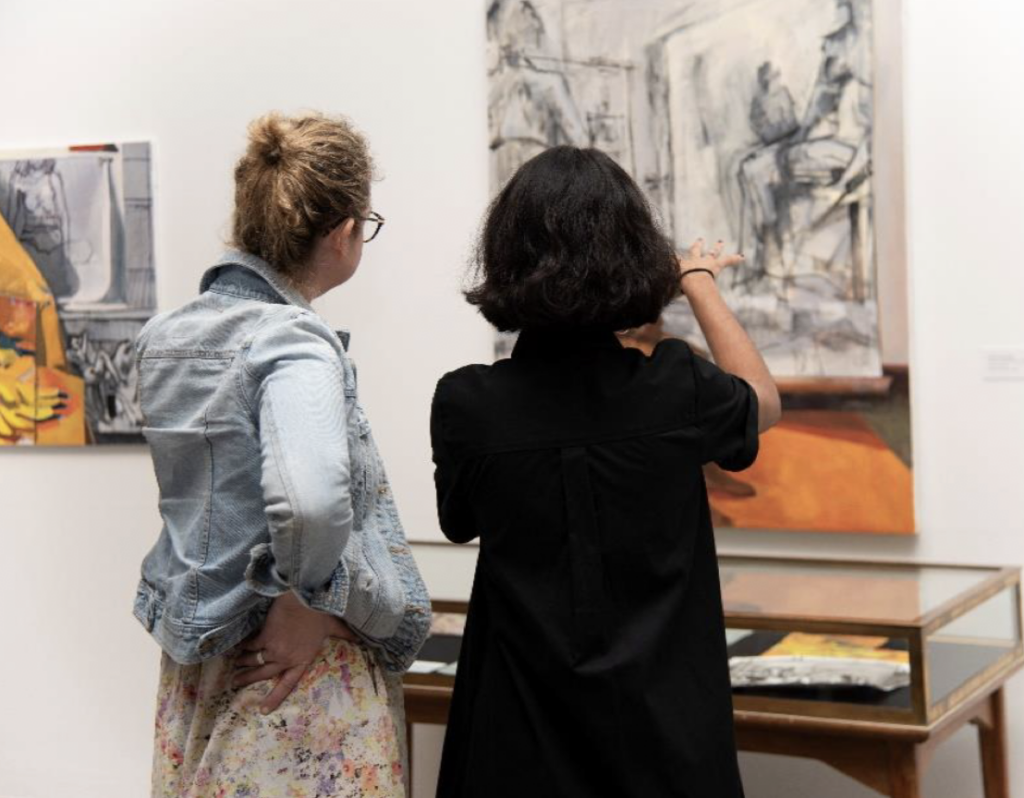This square-shaped photograph appears to be taken in a museum, showcasing two women engrossed in conversation about artwork. Both women are seen from behind, focusing on a black and white charcoal drawing on the plain white wall before them. The woman on the right has dark, short, wavy hair and is dressed in a black shirt or dress. She extends her hand towards the artwork, pointing out its details. To her left stands a woman with light brown hair styled in a bun. She wears a light blue jean jacket over a flowery dress and has her hand poised on her hip. A wooden-framed glass display table filled with papers sits beneath the charcoal drawing. Beside the featured drawing, there is another artwork with hints of orange, yellow, and black. The overall ambiance, underscored by the white walls and detailed exhibits, strongly suggests a museum setting.